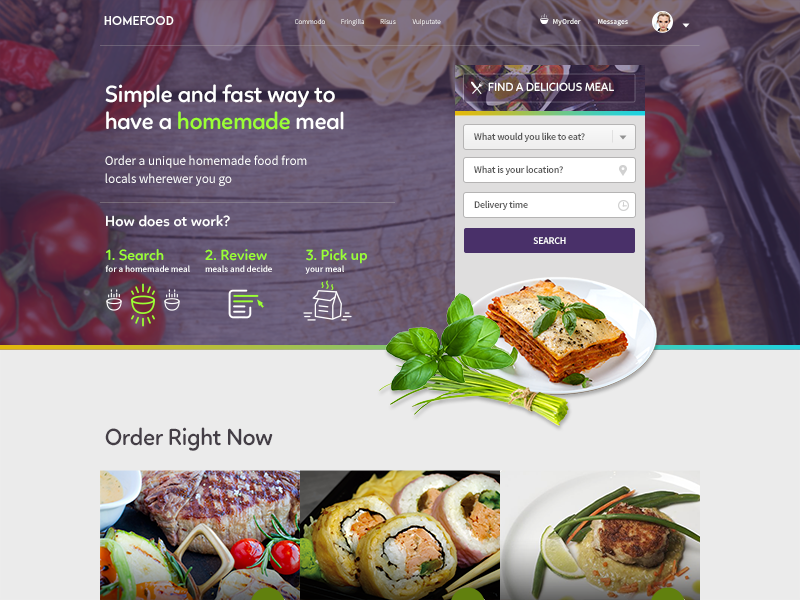**Home Food Website Home Screen**

The home screen of the *Home Food* website, a platform dedicated to providing unique homemade meals from local cooks, features a user-friendly and visually appealing layout. 

**Header Section:**
At the top, the navigation bar in white print includes clickable areas labeled: 

- Fringe Like
- Rhesus
- Volpato
- Commode
- My Order
- Messages

**Background:**
The background gives a warm, inviting kitchen ambiance, showcasing elements like:

- A wooden table or cutting board.
- Fresh cherry tomatoes and peppers.
- Pieces of garlic, both fresh and roasted.
- Various herbs scattered around, enhancing the homely feel.

**Central Content:**
On the left side of the screen, a prominent message reads: 

*"Simple and fast way to have a homemade meal. Order unique homemade food from locals wherever you go."*

Below this, the process is succinctly explained in three steps:

1. Search
2. Review
3. Pick Up

**Search Feature:**
Centrally positioned is a search area prompting users to input:

- Desired food
- Location
- Delivery time

A search button is available for users to start their query.

**Visual Elements:**
- At the forefront, a plate with a tempting slice of lasagna garnished with basil sits prominently.
- To the left, fresh basil stalks complement the dish visually.
- At the bottom, a call-to-action button reads *"Order Right Now,"* accompanied by images of sushi and other meal options.

This detailed and organized layout ensures users can easily navigate and understand how to utilize the *Home Food* platform to enjoy delicious homemade meals.